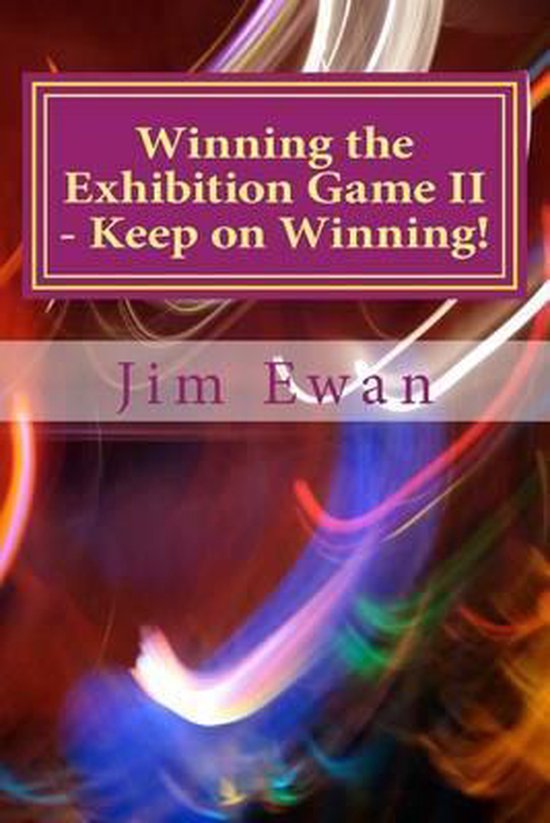This image features a vibrant and dynamic book cover. The predominantly red background is accentuated with various swirling patterns in white, blue, red, and other colorful lines, giving it a celebratory feel. At the top, there's a maroon box with a yellow border, containing the title in yellow font: "Winning the Exhibition Game 2! Keep on Winning!" Below it, a long, skinny, opaque white rectangle showcases the author's name, Jim Ewan, in pinkish-red text. The bottom right corner of the cover displays an orange-yellow smear, resembling a flame, which adds to the overall energetic design. The cover attributes a sense of motivation and triumph, reflecting the themes of the book.